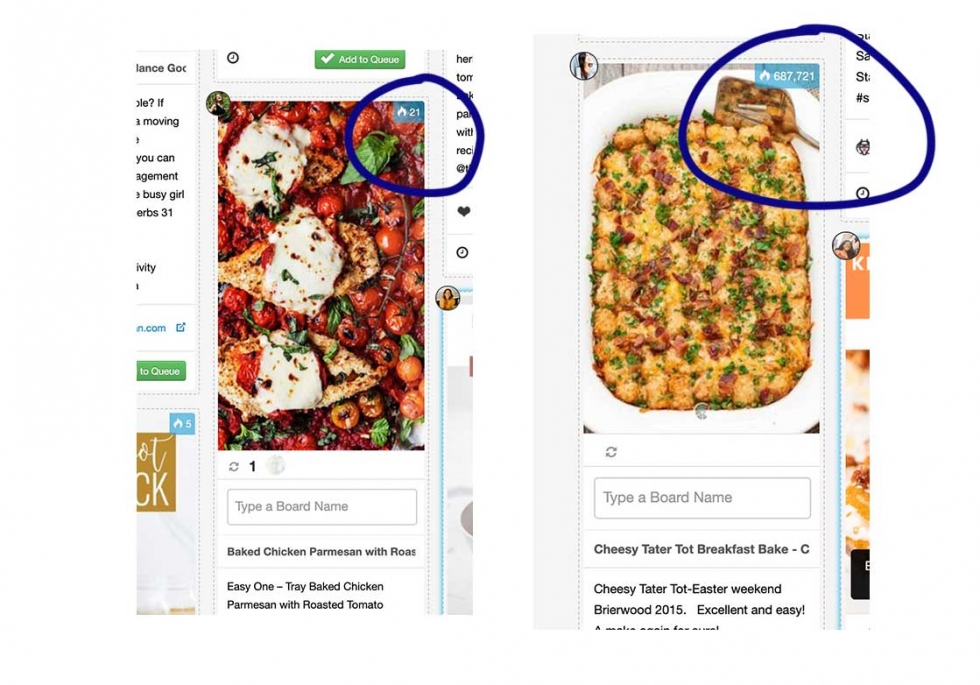**Caption:**

The image showcases a split-screen view, featuring two distinct photographs of meals sourced from a phone. On the left side, the upper photo displays a delicious meal, highlighted by the number "21" within a blue circle situated in the top corner. Below this image, there's a text area with the placeholder "Type a board's name". Underneath the text input, a partial description reads “baked chicken parmesan with R-O-A-S” followed by a recommendation for “easy one, try baked chicken parmesan with roasted tomato.”

On the right side of the split screen, another appetizing meal is presented with the number "687721" prominently circled in the top corner. Beneath this photo, a caption reads "cheesy tater tot breakfast bake," accompanied by the enthusiastic endorsement, "cheesy tater tot Easter weekend, excellent and easy!" 

Both images are neatly annotated with circled numbers and enticing descriptions, offering a glimpse into two distinct yet equally appealing culinary creations.